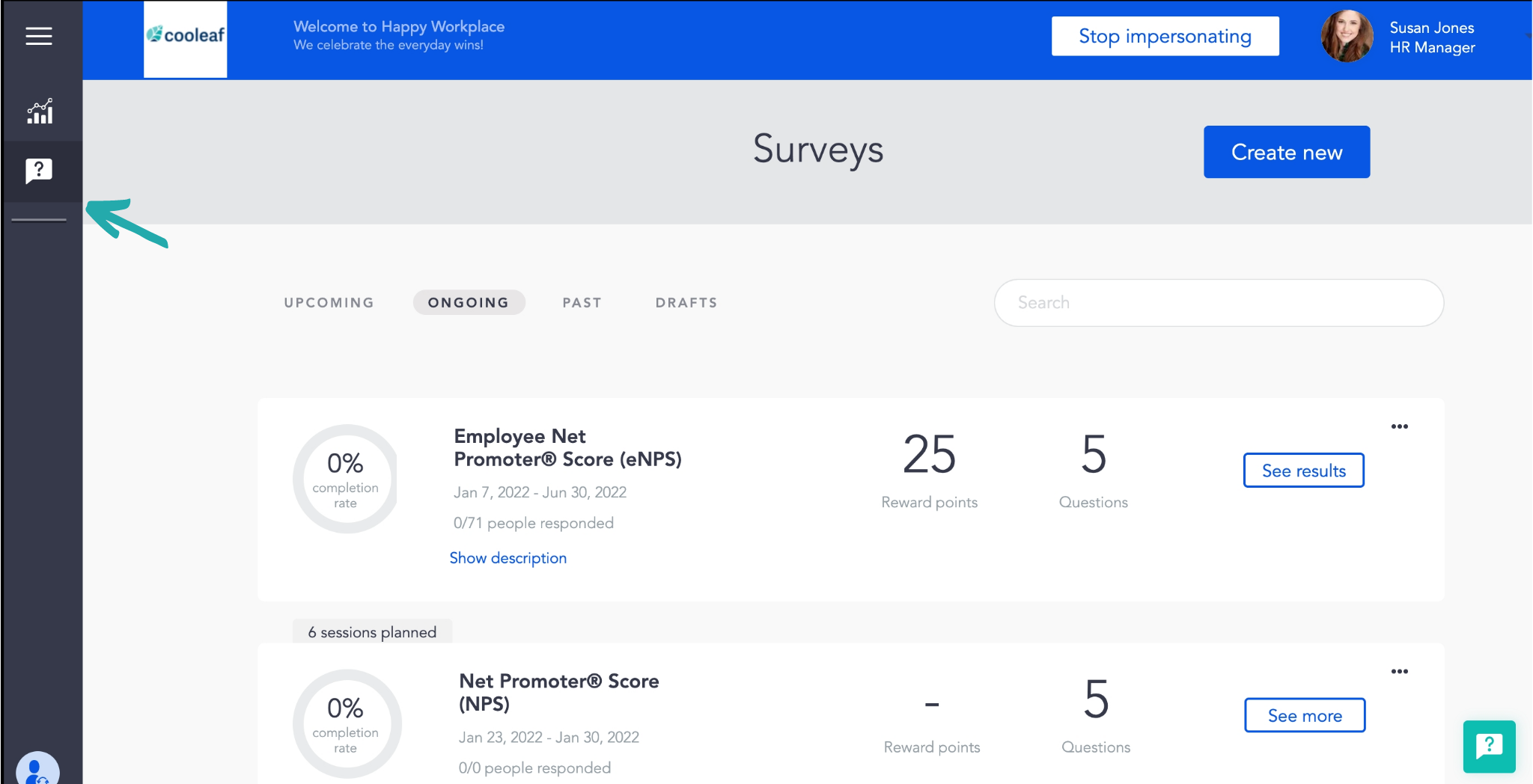This screenshot appears to be a mock-up of a website called "CoolLeaf," identifiable by its title written in bold letters, "C-O-O-L-E-A-F," and a small green leaf icon adjacent to it. The interface features a vibrant blue bar at the top, branding the site with "Welcome to Happy Workplace," though part of the tagline is unreadable. To the right of this banner is a text field labeled "Stop Impersonating" with a possible button beneath it labeled "Create New."

On the left side of the screen, a dark gray menu extends vertically. At the very top of this menu is a hamburger icon, followed by a graph bar icon, and a speech bubble containing a question mark, the latter of which is highlighted by a hand-drawn green arrow pointing directly at it.

Susan Jones, identified as the HR Manager, is displayed with a profile picture prominently on the screen. Below her profile information is a section labeled "Surveys," which includes options for "Create New," "Upcoming and Ongoing," and "Past Drafts."

The "Ongoing" section is further detailed with two survey tiles, both currently showing a 0% completion rate. The first survey is titled "Employee Net Promoter Score," offering 25 reward points for completion, consisting of 5 questions, and includes a "See Results" link. The second survey is titled simply "Net Promoter Score (NPS)," offering no reward points, also consisting of 5 questions, with a link labeled "See More."